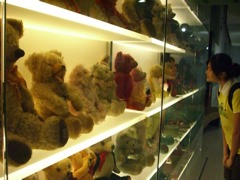This color photo captures a young Asian woman wearing a yellow shirt as she gazes intently at a glass case filled with teddy bears. The glass display, reminiscent of a museum exhibit rather than a store display, houses multiple rows of seated teddy bears arranged on white, fully-lit shelves. These bears, predominantly in shades of light tan and dark brown, vary in size and condition, with some appearing older and a little worn. The shelves are illuminated with an unnatural yellow backlighting, enhancing the visibility of the bears. The glass case's lighting setup includes lights both at the top and bottom of the shelves, ensuring each bear is fully visible. The scene is indoors, with a soft, ambient yellow glow pervading the image.